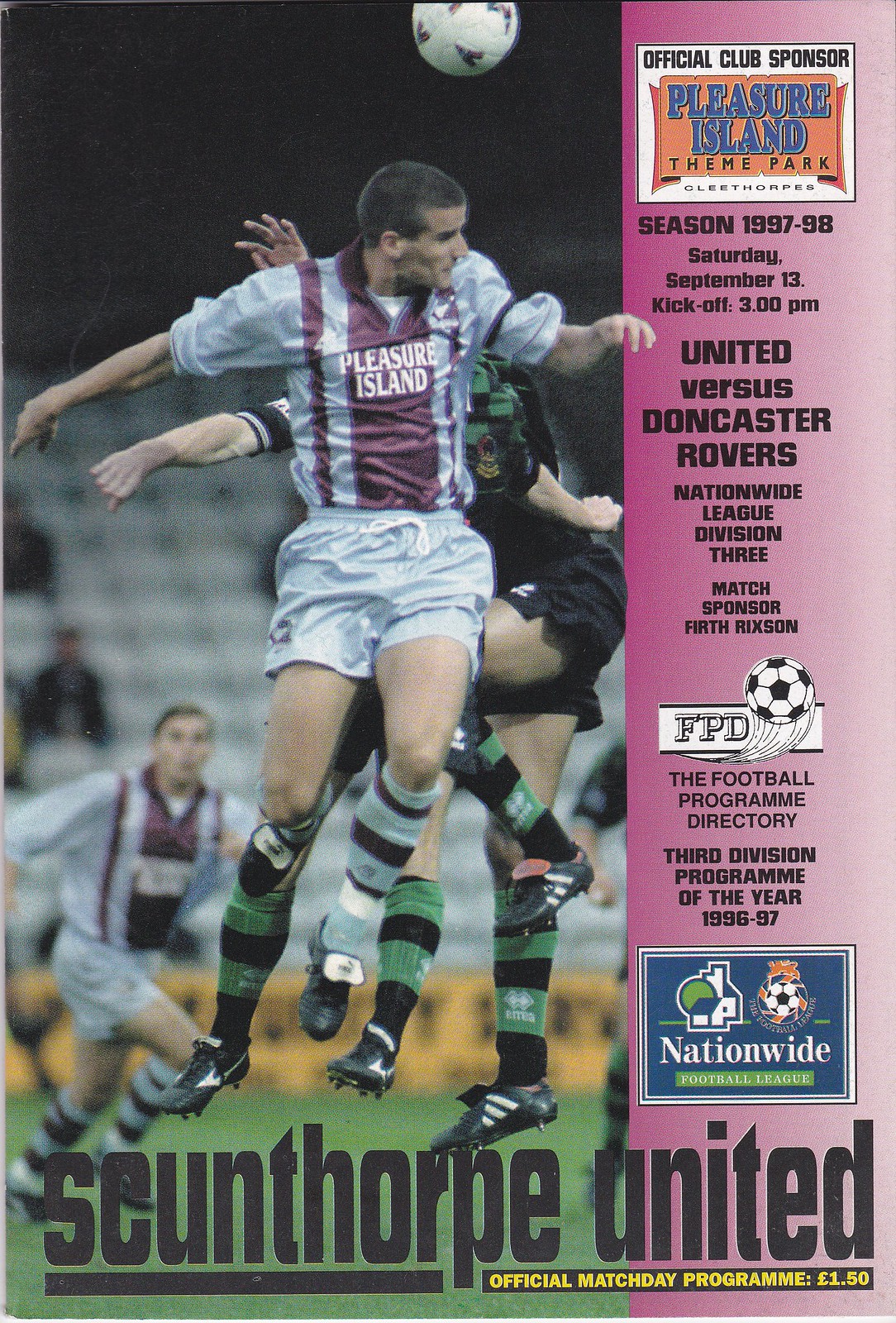The image is a detailed poster for a soccer match between Skunthorpe United and Doncaster Rovers, part of the 1997-98 Nationwide League Division III season. The poster prominently features a background photo of a game in progress where a player in a purple and blue striped uniform, sponsored by Pleasure Island, leaps to head the ball. Another player in a green and black uniform defends in the background. The text on the right side of the poster lists various details including: "Skunthorpe United Official Match Day Program" at the bottom, the cost of the program which is 1.5 pounds, and information about the match including the date, Saturday, September 13th, and the kickoff time of 3 p.m. The poster also features logos for the club and the Nationwide League, as well as a smaller text noting "Third Division Programmer of the Year." It serves as both an announcement and a program guide for the matchday event.